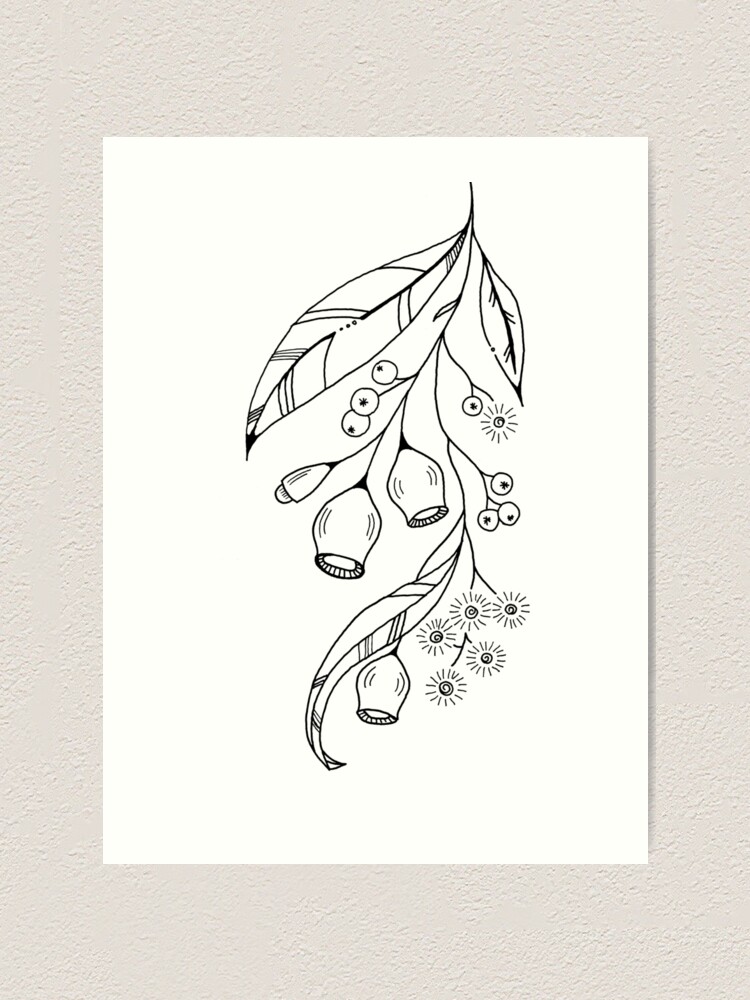This vertical rectangular image features a detailed pen and ink drawing of a plant with various leaves and blossoms. The drawing, upside down, places the stem at the top and the blossoms at the bottom, with a pointed leaf extending furthest down. The artwork, rendered on white paper and matted with a grayish border, showcases at least two, likely three, different types of flowers. The leaves are intricately detailed with channels and pointed tips, while the blossoms exhibit finely drawn petals. The entire piece, created using black ink, appears to use pens of varying sizes for detailed emphasis. The drawing is mounted on a beige wall, suggesting it is displayed as part of an exhibition.